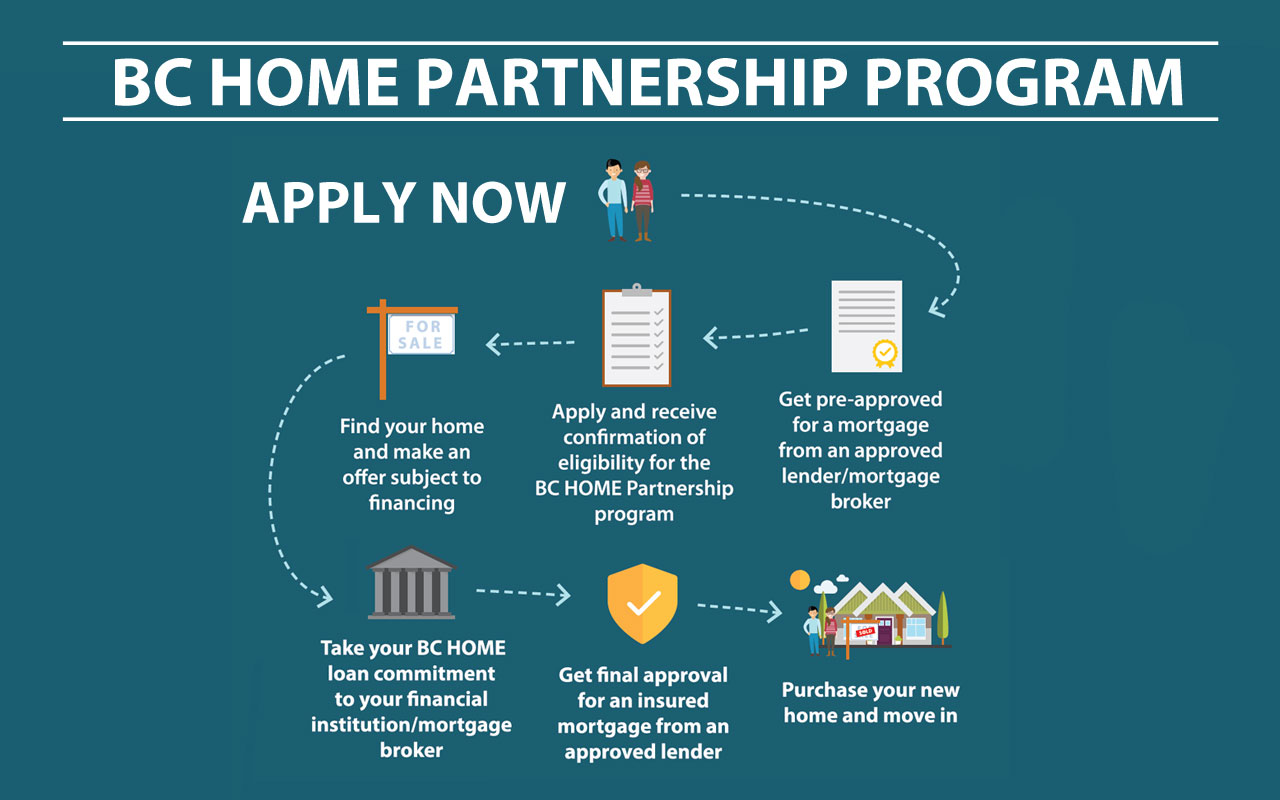The image is an informational graphic design advertisement for the BC Home Partnership Program. The background is a dark teal color with bold white text at the top stating, "BC Home Partnership Program," flanked by horizontal white lines. Directly below this title, on the left side, is the call to action "Apply Now" in bold white text. The central part of the image contains a detailed, step-by-step guide to applying for the program, arranged in two rows of three illustrated steps each, connected by dotted arrows.

The steps are visually represented with small color illustrations and accompanying text descriptions. The first row, from right to left, includes a piece of paper, a clipboard, and a "For Sale" sign, marking the initial steps: getting approved for a mortgage from an approved lender or mortgage broker, applying for the program, and receiving confirmation of eligibility. The second row, from left to right, depicts a courthouse, a shield with a check mark, and a house, illustrating the subsequent steps: finding a home and making an offer subject to financing, committing to the BC Home Loan with your financial institution, receiving final approval for an insured mortgage, and finally purchasing the home and moving in. 

The color palette includes browns, whites, grays, golds, greens, and touches of magenta to position the various objects and text, all harmoniously integrated into the digital graphic. This image effectively guides viewers through the application and approval process for the BC Home Partnership Program, using a blend of graphic design, color illustration, and clear typography.